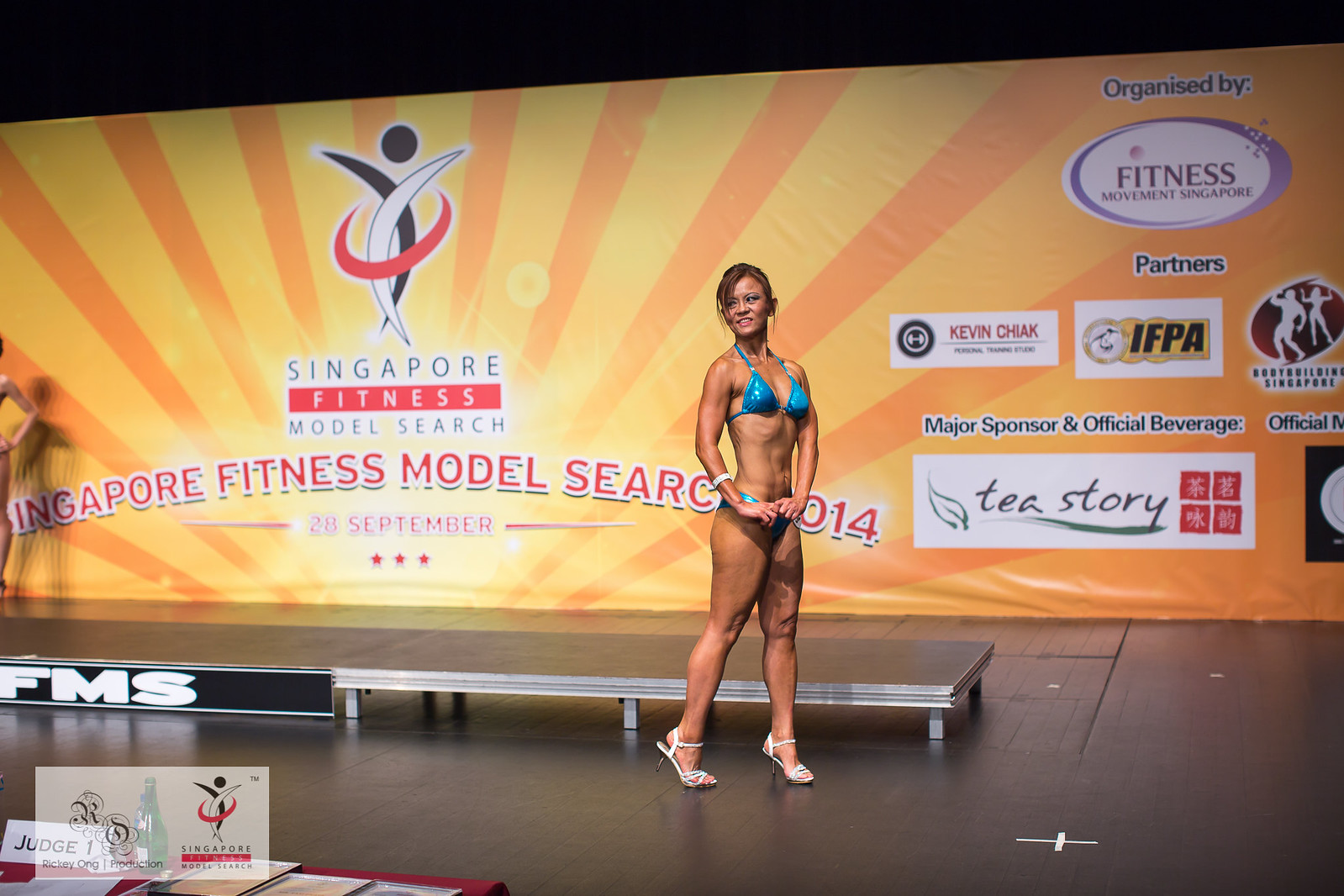In this image, a female fitness model is competing in the Singapore Fitness Model Search 2014. She is confidently standing and posing on stage, looking away from the camera. She wears a striking blue bikini paired with white high-heeled shoes. Behind her, a billboard displays the text "Singapore Fitness Model Search" alongside advertisements from various companies, featuring a color palette that includes orange, white, and aqua blue. The setting appears to be a convention center or an auditorium, specifically designed with a stage to host the competition.